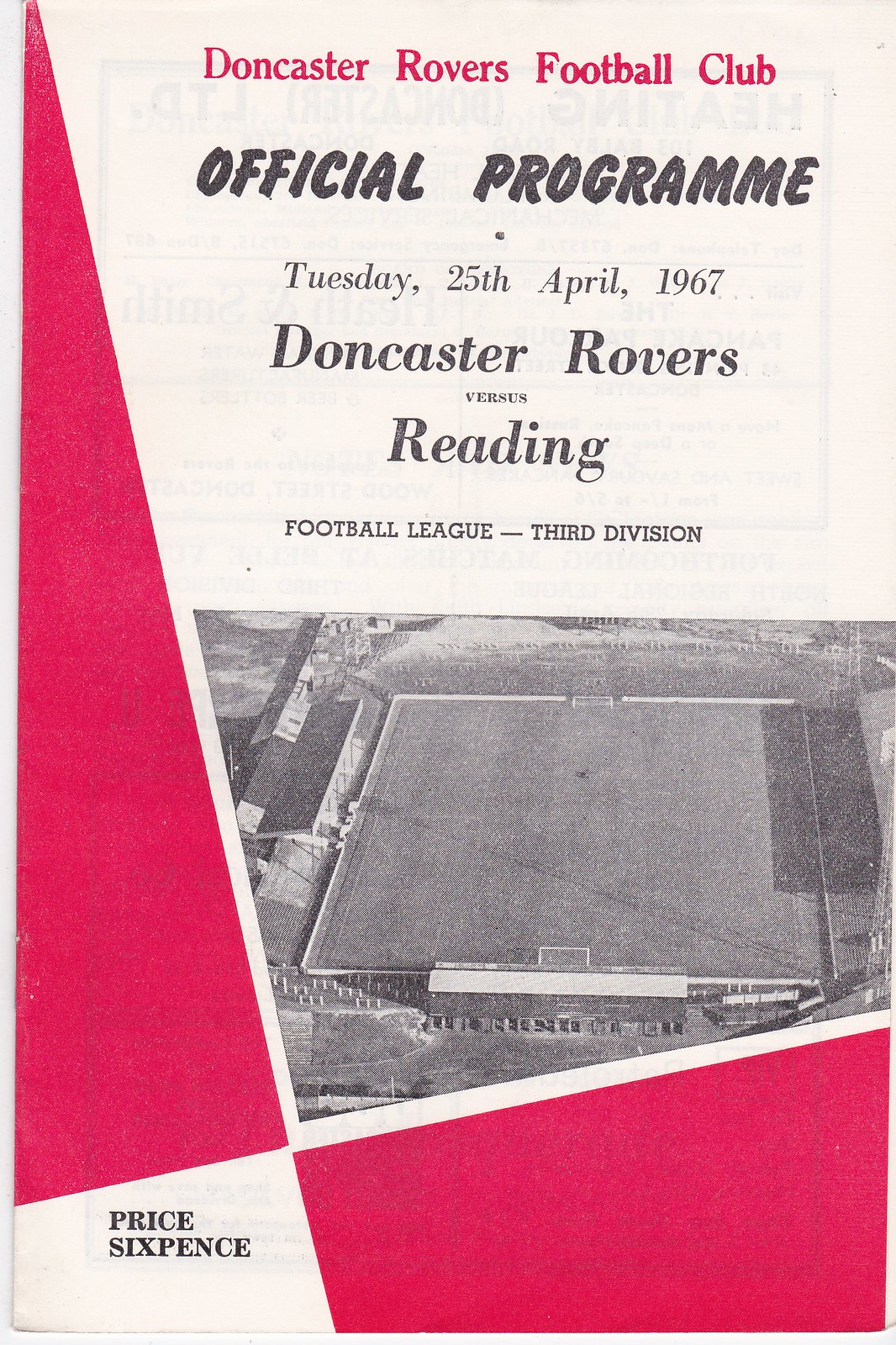This image shows the front cover of an official program for the Doncaster Rovers Football Club, dated Tuesday, April 25th, 1967. The program, priced at six pence, is from a match in the Football League Third Division where Doncaster Rovers faced Reading. The cover features a red and white design with a distinctive hot pink triangle graphic that extends across the left to right side. In the center, there is a black-and-white aerial photograph of the playing field, surrounded by buildings and bleachers. The text on top reads "Doncaster Rovers Football Club Official Program," detailing the event specifics and highlighting its vintage charm from the sixties.